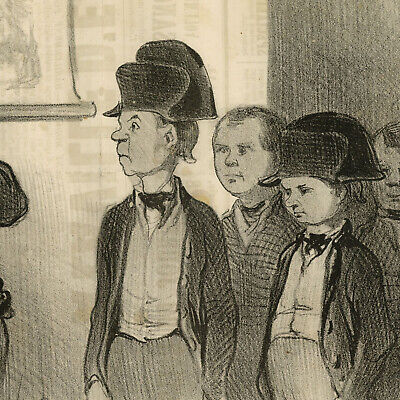The black and white pencil drawing vividly illustrates four characters with a blend of cartoonish and realistic features, suggesting an old European influence. The figures have round faces and slender bodies, all dressed in jackets, vests, long coats, and pants. Two characters at the front don Russian-style hats, while the two behind them are hatless. They all exhibit bothered or upset expressions as they stand facing left in an interior space.

The background features a white wall with intricate hatch marks and texture, creating depth with patterns of lines. A partially visible painting or piece of paper is mounted on the upper left side of the wall. The left section of the image has some portions cut off, revealing a dark-colored round mound and another indistinct object near the bottom. The meticulous pencil work emphasizes the clear and detailed quality of the drawing, devoid of any textual elements, capturing the viewers' attention with its precise natural lighting and stark contrasts.